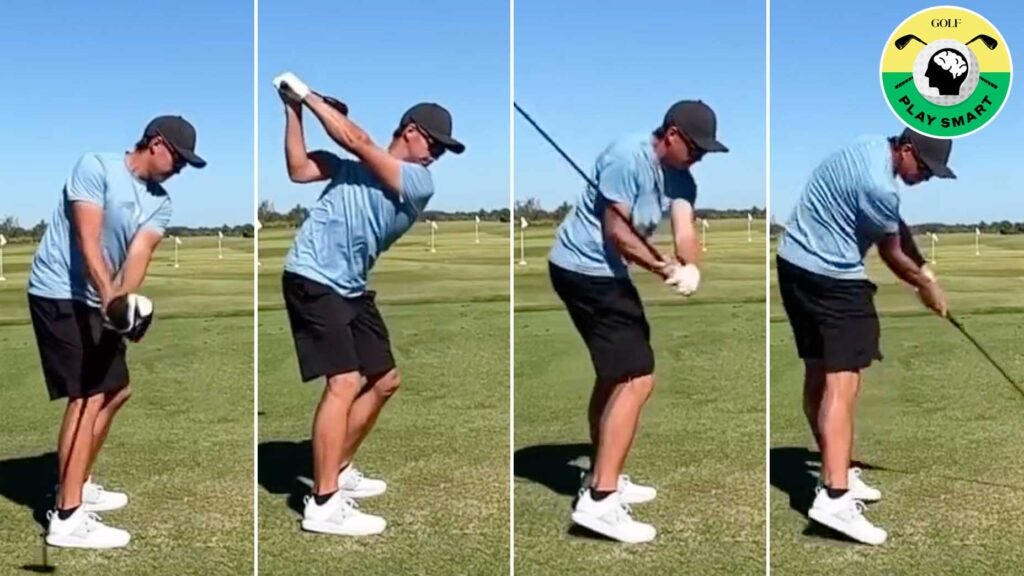The image is a mosaic featuring four vertical photos, capturing the sequential progress of a man’s golf swing, from left to right. The man is outdoors on a bright and clear day, evident by the light blue sky with no clouds in sight. In the background, a horizon line of green trees and smooth light green grass typical of a golf course is visible, along with distant white flags. The golfer is consistently dressed in a black baseball hat, light blue t-shirt, black shorts, white shoes, and black socks. In the first photo, the man is poised with the golf club next to the ground, preparing for the swing. The second photo captures the club raised near his neck, held at the peak of his backswing. The third photo shows the golfer in mid-swing, with dynamic motion evident. The final photo depicts the moment of impact where the club hits the ball, with visible movement in his feet. The upper right corner of the image features a detailed logo for "Golf Play Smart," which includes a brain with two crossed golf clubs and a golf ball inside a circular design, with colors transitioning from yellow at the top to green at the bottom.